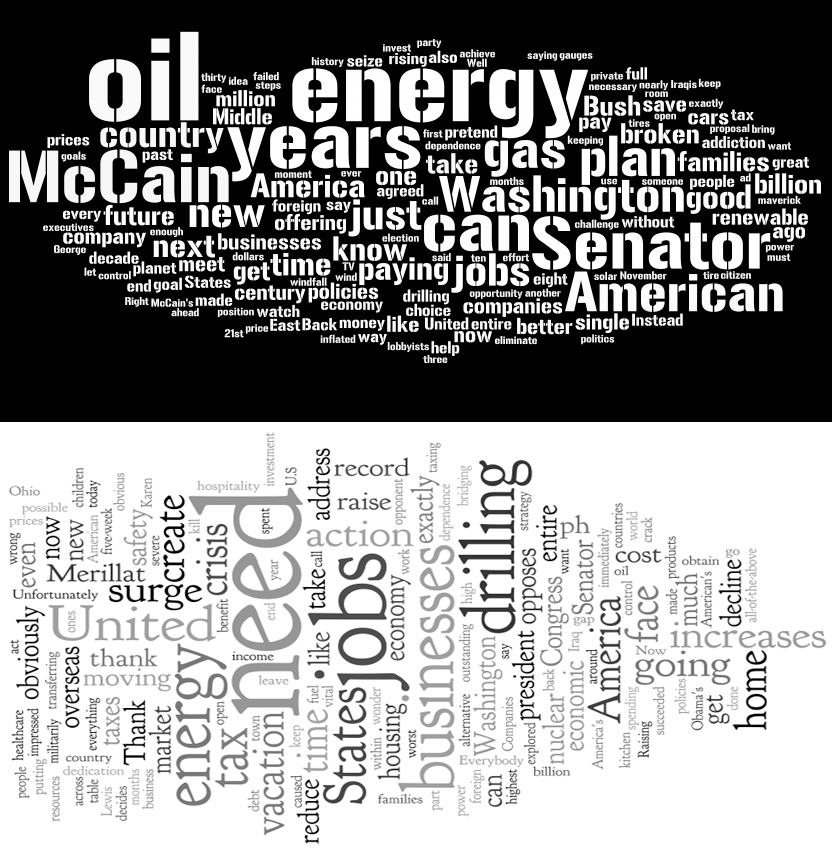This digital image features a striking black and white word collage that juxtaposes two distinct halves. The top half showcases a black background peppered with words in stark white text, emphasizing terms like "Oil," "Energy," "Years," "Gas," "Plane," "Washington," "Senator," "American," "McCain," and "New" in varying font sizes, creating a dynamic visual hierarchy. Smaller words such as "Lobbyists," "Three," "Help," "Politics," "Keep," and "Iraqis" nestle among the larger ones, adding depth and complexity.

In contrast, the bottom half boasts a white background with a mix of horizontally and vertically aligned words in shades of gray. Here, prominent words like "Need," "Jobs," "Drilling," "Business," and "America" dominate the space, while smaller words like "Raising," "Oil," "Crack," "US," and "Unfortunately" provide nuanced details. This half also includes terms like "Home," "Going," "Increases," "Search," "Marillat," and "Create," further enriching the collage. The overall arrangement forms a squat pumpkin shape when viewed from afar, crafting a visually intricate narrative that contrasts the perceived negativity of the top half with the seemingly more positive undertones of the bottom half.